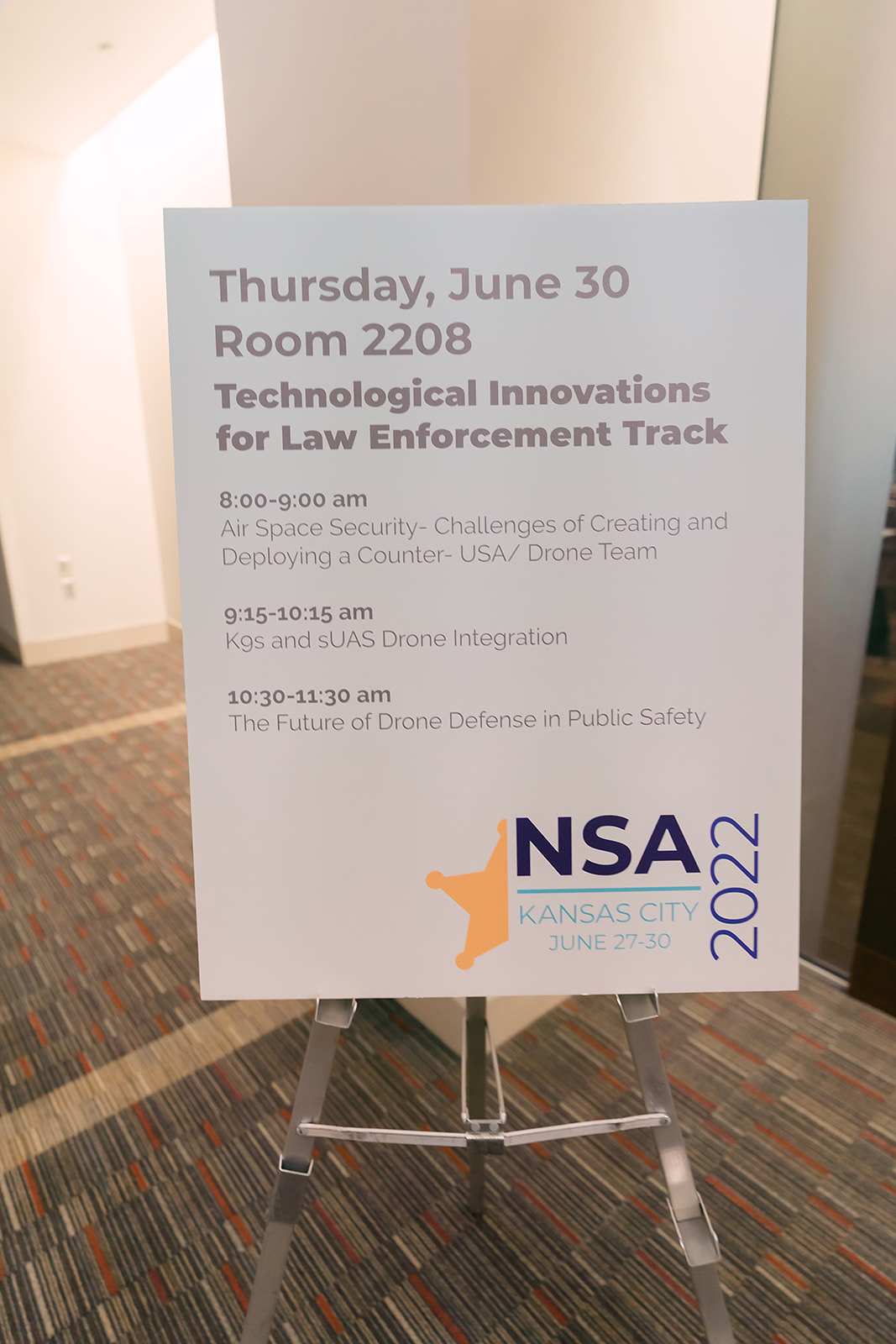The image depicts a large white poster board sign mounted on a silver metal easel. The sign is positioned on a patterned carpet with black, white, and red stripes, suggesting it is placed in the lobby of a hotel with white walls. The sign details a conference schedule for "Technological Innovations for Law Enforcement Track," taking place on Thursday, June 30th, in room 2208. The conference sessions include "Airspace Security: Challenges of Creating and Deploying a Counter-USA/Drone Team" from 8 to 9 a.m., "K-9s and SUAS Drone Integration" from 9:15 to 10:15 a.m., and "The Future of Drone Defense and Public Safety" from 10:30 to 11:30 a.m. The event is sponsored by NSA Kansas City and spans from June 27th to 30th, 2022. The poster also features a partial gold star logo icon in the background.